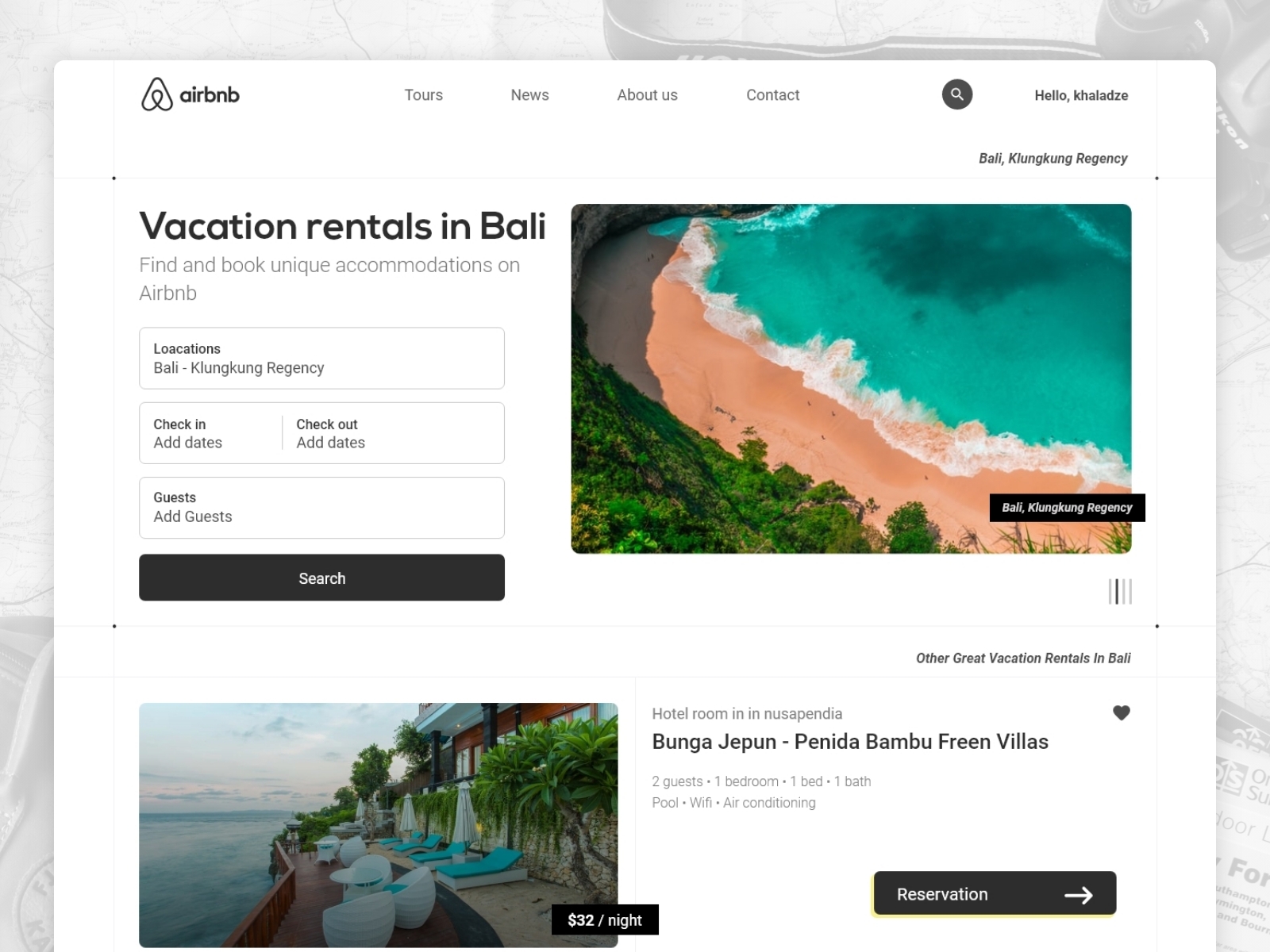This is a detailed screenshot from the Airbnb website displaying a clean and modern pop-up interface. The background features a barely discernible gray marbleized pattern, creating a sophisticated contrast to the prominent white pop-up box in the foreground.

At the top left corner of the white box, the unmistakable Airbnb logo is displayed. Below the logo, there are four hyperlinks: "Tours," "News," "About Us," and "Contact." On the right side of this upper section, a search bar is visible alongside a greeting, "Hello, KHALADZE."

Beneath these, a section titled "Vacation Rentals in Bali" invites users to "Find and book unique accommodations on Airbnb." This section includes four input fields for location, check-in and check-out dates, and number of guests, followed by a prominent search button.

To the right of the input fields, there's an overhead, macro view of a picturesque beach with vivid blue waters, tan sand, and lush tropical foliage, labeled as "Bali Kang Regency."

In the lower quadrant of the interface, another image showcases a striking hotel built atop the ocean on a jetty. This scene features lounge chairs, surrounding foliage, retainer walls, and structures with orange siding. The text below the image identifies the hotel as "Nusa Penida, Bangai, Jepun, Pinda, Bamboo Green Villas," accommodating two guests with one bedroom, one bed, one bath, no pool, Wi-Fi, and air conditioning, all for $32 per night. A booking button is conveniently placed for users interested in reserving this particular location.